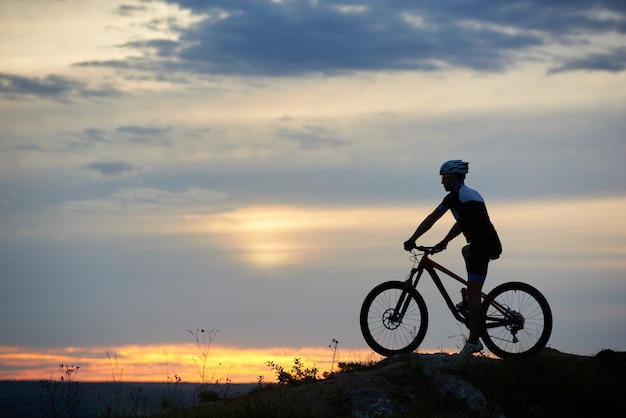In this evocative photograph capturing a serene moment at sunset, we see a cyclist, clad in a black and light blue biking outfit with a helmet, stopped on a rugged hillside. The cyclist's black mountain bike rests beneath him as he gazes out towards the mesmerizing horizon. His right foot remains poised on the pedal, while his left foot stabilizes him on the ground. Sparse and scrubby vegetation sporadically dots the foreground, further enriching the scene's rustic charm. 

The sky dominates the image, transitioning from a warm yellow and orange glow near the horizon—which could hint at either sunrise or sunset—to lighter shades of gray and hints of purple as it stretches upward, interspersed with wispy and denser gray clouds. A slight opening allows a glimpse of lighter purplish-gray hues on the left. Far in the distance, the blurred silhouettes of sparse trees and elongated shadows add depth, reinforcing the tranquility and expansive feel of this outdoor setting, possibly overlooking the ocean. Overall, the scene captures a powerful, meditative moment of a man and nature in harmonious stillness.